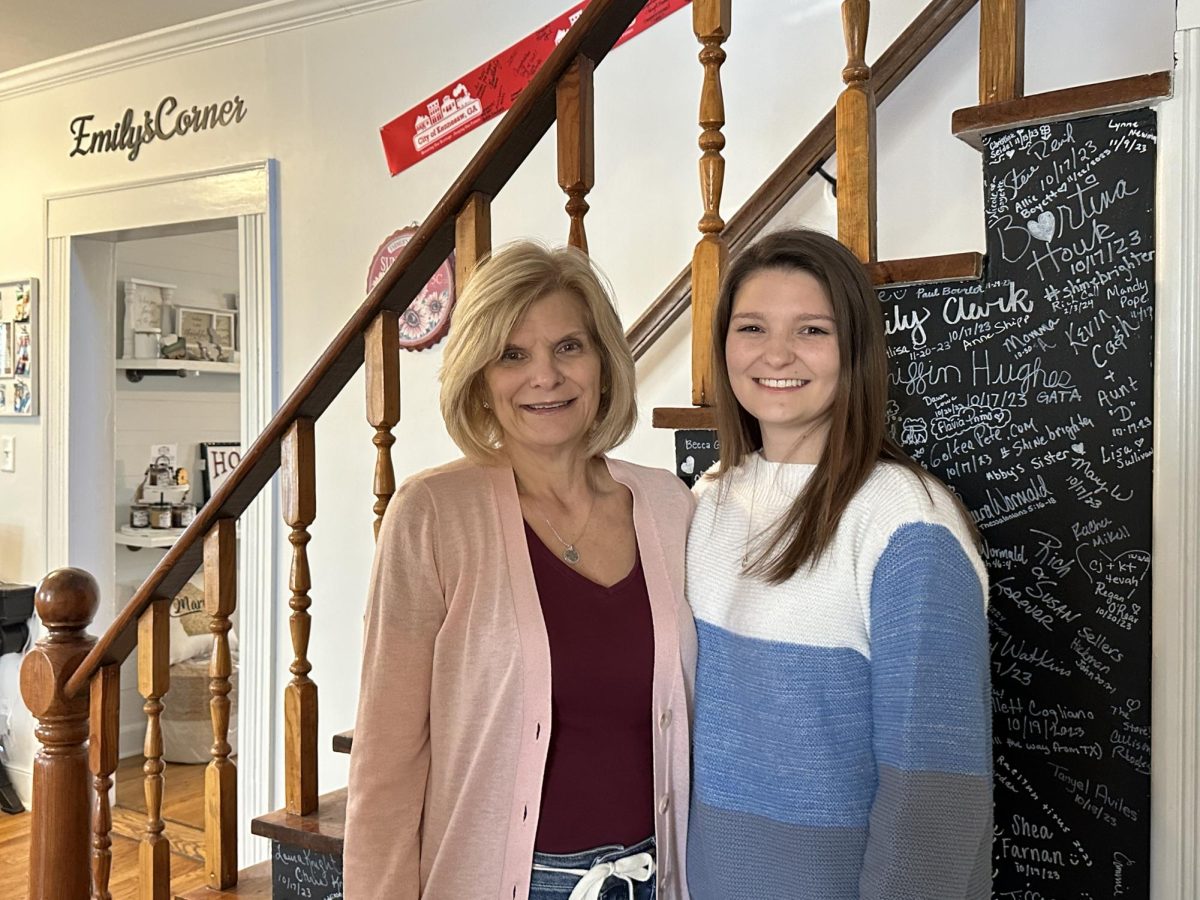In the image, two females, likely a mother and daughter, are standing in front of a black-painted staircase adorned with white chalk writings. The older female, presumed to be the mother, has short blonde hair, and is dressed in a pink coat over a purple shirt, blue jeans, and a white belt. The younger female, likely the daughter, has long dark hair and is wearing a white, blue, and gray long-sleeved shirt, smiling. Behind them, the stair posts and ledge railings are made of brown wood, and the walls are white. Above a doorway to their left, the words "Emily's Corner" are displayed in black text. Inside this adjacent room, which resembles a pastry or kitchen retail area, the decor features white walls, silver and black picture frames, and candles on white shelves. Scattered white text on the black chalkboard behind the staircase includes various names and phrases, adding a personalized touch to the setting. Additionally, there is a black table in the bottom left of the picture, and the floor appears to be brown. The scene suggests a cozy, family-friendly environment, possibly part of an exhibit or shop.